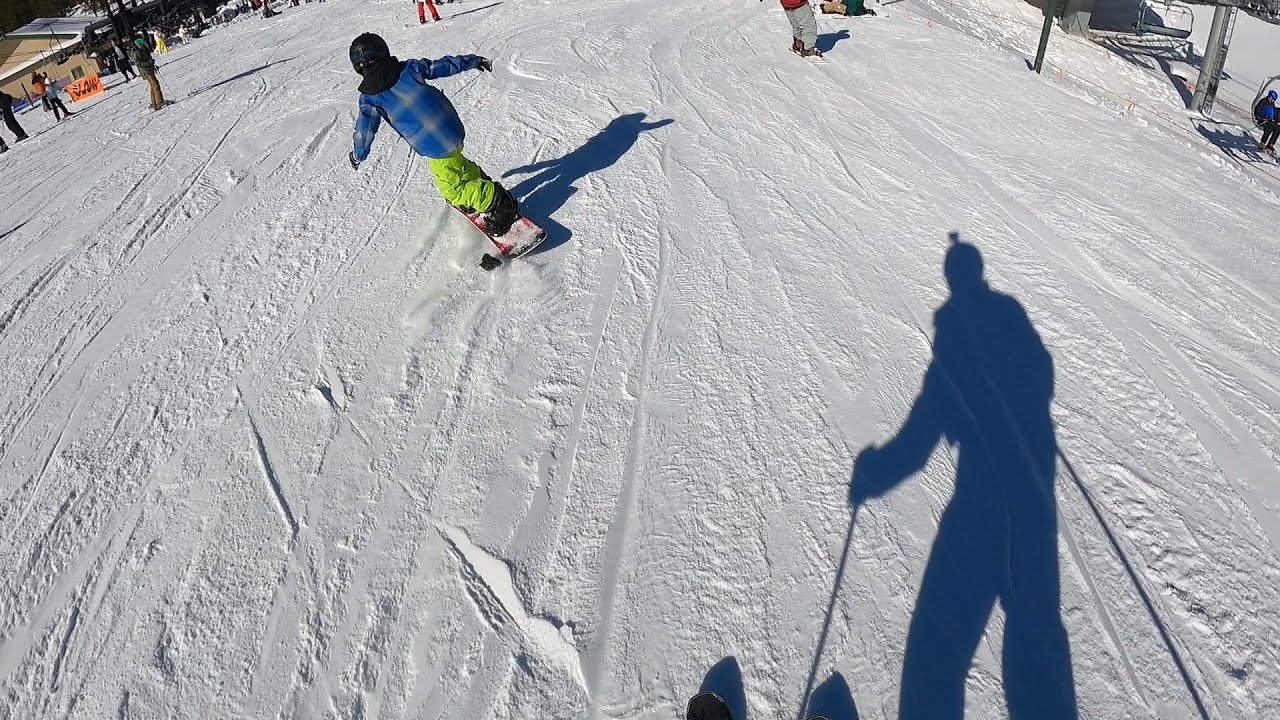The image is a vivid first-person view from the vantage point of a skier, captured by a helmet camera, possibly a GoPro. The skier's shadow, along with the shadows of their ski poles, is prominently displayed on the pristine, snow-covered ground. Directly ahead, a child in light green pants, a blue coat, and a helmet is snowboarding. The background reveals a bustling ski resort with several indistinct figures further away, all engaged in skiing or snowboarding activities. To the left, there's a small building with an orange sign, and on the right, portions of a ski lift are visible. The snowy landscape is marked by numerous ski and snowboard tracks, with colors ranging from blue, yellow, and red to more neutral shades like gray, tan, brown, and silver. The sun is behind the skier, casting all the shadows towards the right-hand side of the image.